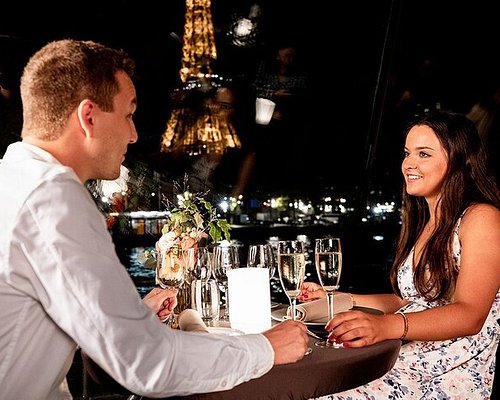In this iconic and romantic scene, a couple in their late 20s is seated at a small round wooden table, engaged in an intimate moment. The man, wearing a gray long-sleeved shirt, is positioned on the left, while the woman, dressed in a white dress with blue and yellow floral embroidery, sits across from him. They both hold champagne glasses, appearing as though they are about to toast, their hands resting gently on the table. The table is adorned with a small bouquet of flowers and set with empty plates, the silverware still wrapped in napkins, indicating that their meal is yet to be served. In the background, the Eiffel Tower is beautifully illuminated against the night sky, with its majestic structure visible up to the midpoint. Streetlights from nearby businesses and buildings add a warm glow to the scene, and a body of water lies between the couple and the iconic landmark, enhancing the romantic atmosphere.